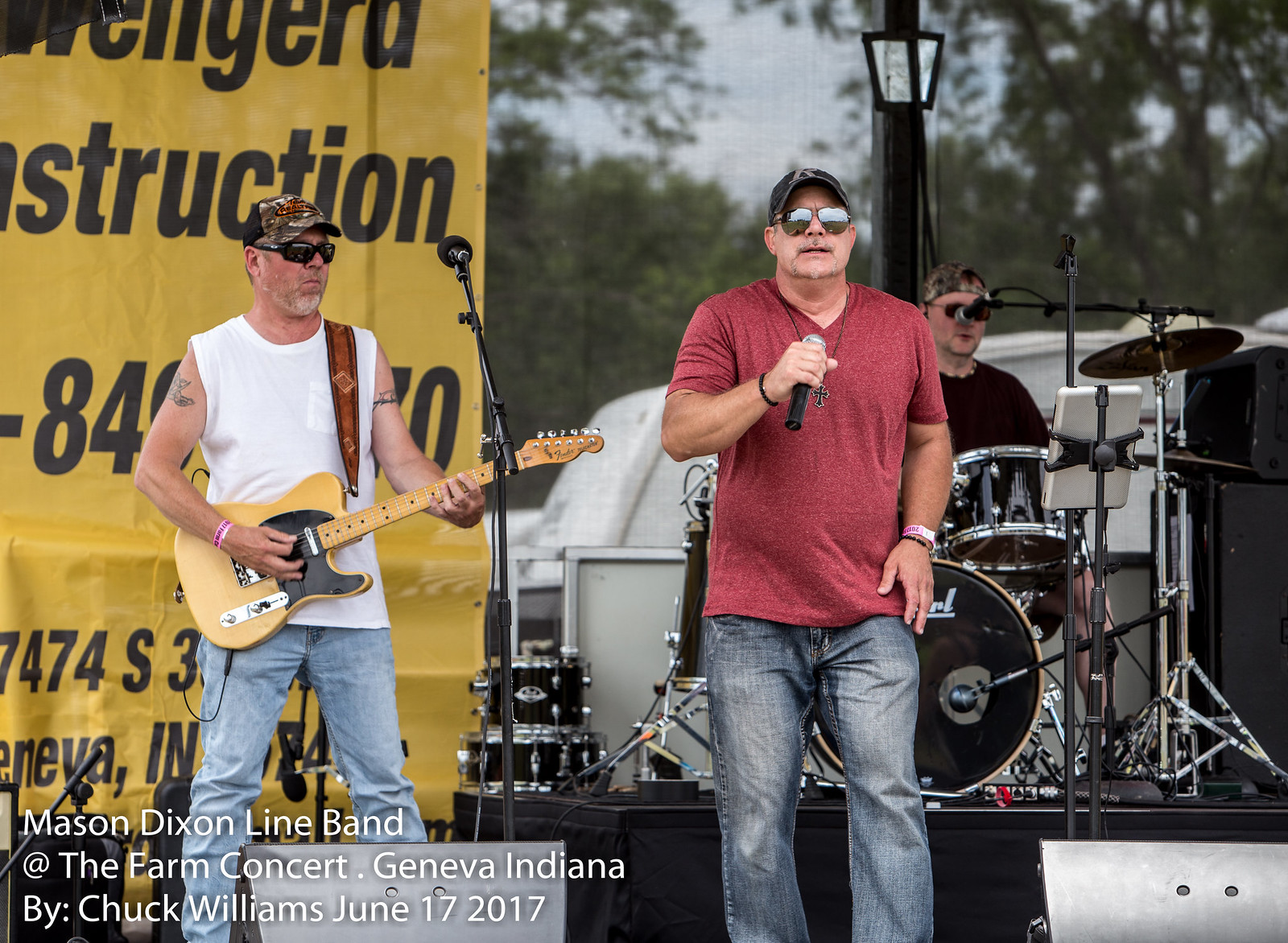The photograph captures an outdoor daytime band performance, with the Mason Dixon Line Band on stage at the Farm Concert in Geneva, Indiana, taken by Chuck Williams on June 17, 2017. Central to the image is the lead singer, wearing a red polo, blue jeans, sunglasses, a black cap, and a cross chain. He is holding a microphone and stands as the focal point. To his right, there is a drummer dressed in a black t-shirt and black backwards cap, positioned behind a drum kit. On the left side of the stage is a guitarist with a white sleeved shirt, blue jeans, a camo cap, sunglasses, and a yellow electric guitar with a brown strap. The stage is set against a backdrop that includes a yellow banner with black text, partially visible on the left. Additionally, the sky and trees are visible behind the stage, framing the performance. The bottom left of the image has a superimposed caption that reads: "Mason Dixon Line Band at the Farm Concert, Geneva, Indiana by Chuck Williams, June 17, 2017."